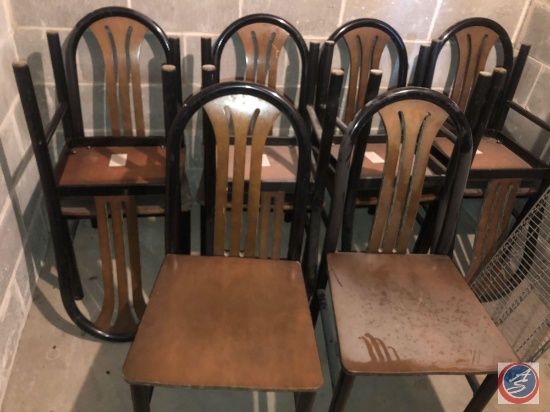The image displays a narrow, basement-like area with cinder block walls, and a stone or cement floor. Scattered amidst this space are ten old and dirty dining chairs, many of which appear to have once been part of a church or similar institution. The chairs feature wood bases, black lacquered frames, and wood insets in the back, and they are arranged in disarray. Some chairs are simply standing, while others are stacked upside down on top of each other, indicating a long period of neglect given the dust covering one of them. A white iron rack leans against the stone wall on the right side, adding to the cluttered feel of the room, which might suggest this space is being used for storage. Labels on the chairs and a text with an “A” on top of an “S” within a red circle and blue background hint at possible advertising for sale or free pickup. The overall scene gives an impression of items long forgotten and awaiting disposal or reclamation.